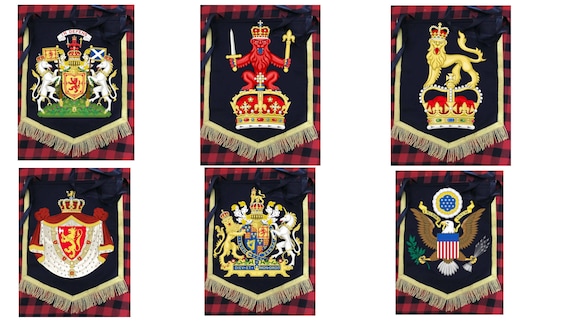The image showcases six embroidered patches, each resembling military or royal insignias, meticulously embroidered on black and red plaid fabric. On the top left, there is a heraldic badge featuring two white horses rearing towards a family seal, exuding an old-fashioned and royal aesthetic. The center top patch displays a red animal, which appears to be a bear, holding a scepter and a sword aloft above a crown. To the right, a yellow lion wearing a crown is majestically perched on another crown. 

At the bottom left, a patch depicts a red flag adorned with a yellow lion also crowned, on a shield. The bottom center reveals a duo of animals: a crowned yellow lion on the left and a rearing white horse on the right, together flanking a central seal. Finally, the bottom right showcases the American national emblem, featuring a bald eagle clutching arrows in one talon and an olive branch in the other, with an American flag in the background. These intricate designs lack textual descriptions but convey a rich sense of historical and symbolic significance.